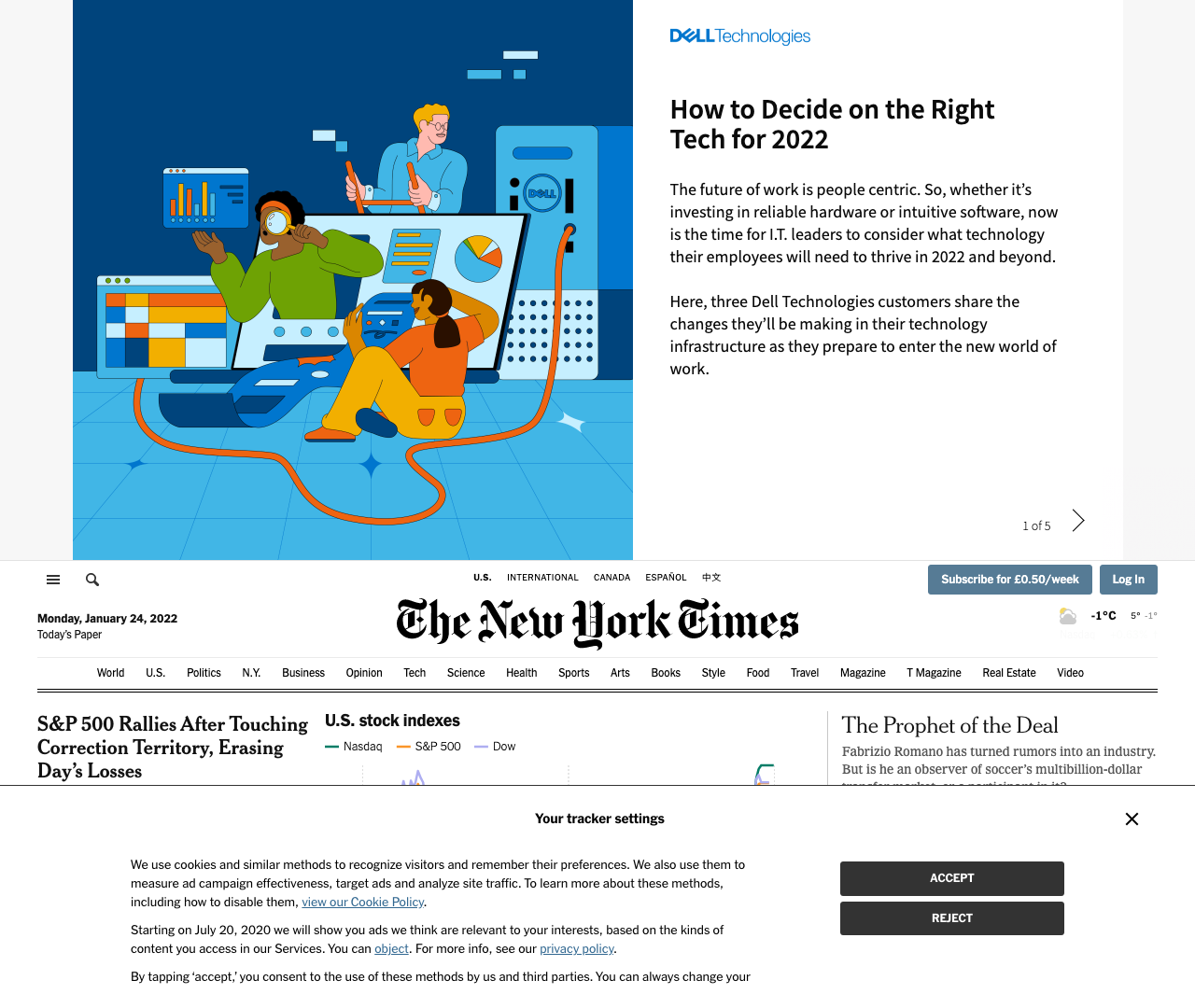The image showcases a screenshot from the New York Times app, specifically displaying a Dell Technologies advertisement. The upper section of the image is dominated by the advertisement, which features a dynamic scene of tech workers engaging with various devices. On the left side, a large box contains two workers: one holding a screen displaying a graph and another sitting on the ground, focused on a machine. In the background, a man stands facing to the left (our right), looking at a Dell machine connected to a monitor with an orange cord. 

To the right of this visual, the text reads, "Dell Technologies: How to Decide on the Right Tech for 2022." The ad emphasizes that the future of work is people-centric, advocating for investment in reliable hardware and intuitive software. It encourages IT leaders to discover the technology their employees need to thrive in 2022 and beyond, highlighting the importance of customer opinions in shaping these decisions.

Below the advertisement, the New York Times UI is visible with some navigational elements. It includes options to access the U.S. edition, international edition, Canada, Espanol, and Chinese editions of the newspaper. There are clearly marked buttons for subscribing at 50 cents per week and logging in. Beneath the New York Times logo, various page categories are listed, allowing users to navigate through different sections of the publication. This content appears to be on page 105, as indicated by an arrow navigation cue.